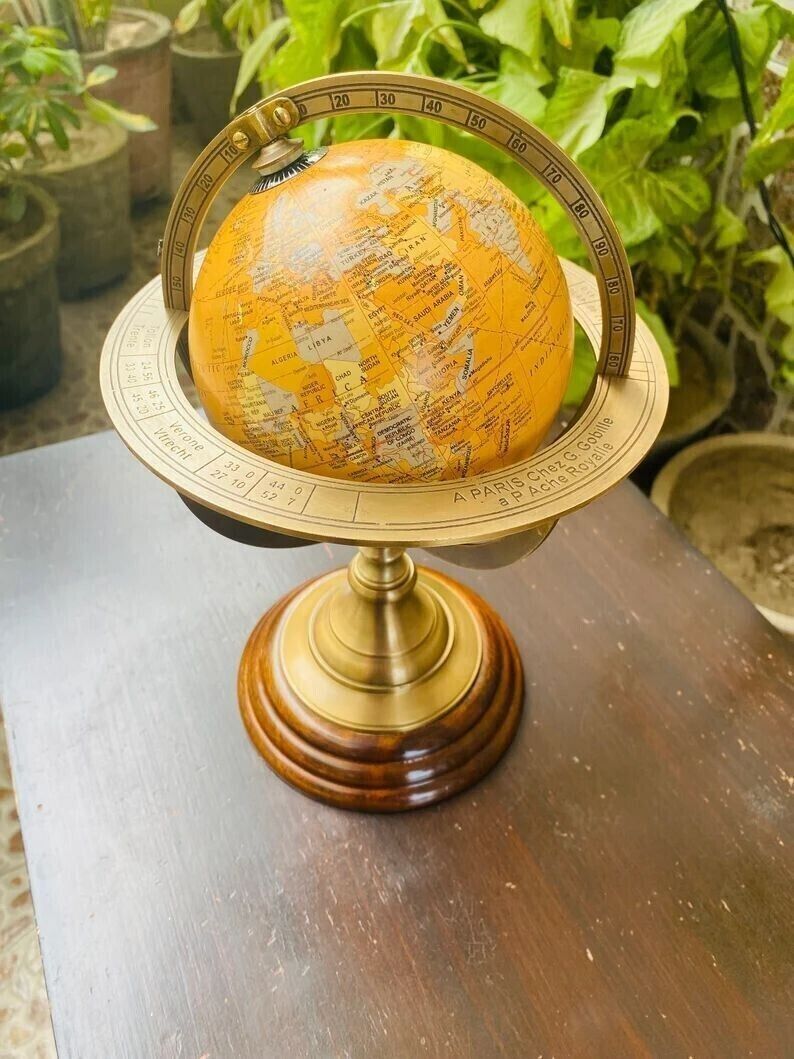This vertical color photograph depicts a globe positioned on a rustic wooden table. The globe, featuring an unconventional color palette with yellows, oranges, tans, and grays where the oceans are represented in yellow, showcases a view of Africa, Asia, Russia, and Europe. It is encased in a brass meridian and an equatorial ring, resembling Saturn's rings, with inscriptions such as "A. Parachay G. Foville" along with various other letters and numbers indicating degrees. A distinctive gold stamp adorns the globe's surface. The base of the globe is a spiral-shaped dark brown platform set upon a flat wooden plank. Surrounding the table are several gray potted plants with light green, lime-colored foliage, adding a natural backdrop to the scene. The photograph is well-lit, bringing sharp focus to the globe's detailed textures and muted hues.